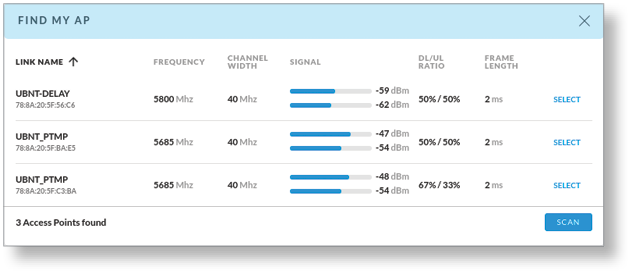The image depicts a pop-up window from a computer application. At the top, there is a light blue header with grey text reading "Find My AP" on the left and a "Close" button on the right. The window has a subtle shadow beneath it, creating a 3D effect.

Within the pop-up, the main content is arranged in a table format against a white background. Near the top, in black text, is the heading "Link Name" with an upward arrow next to it, indicating that the list is sorted by this column. Below this heading, three link names are listed: "UBN", "T Delay", and others.

Further columns display various technical details:
- A list of identifiers organized into groups, such as "UBN TPTMP" followed by numbers.
- Frequency values for each link: 0.800 MHz, 5.685 MHz, and 5.685 MHz.
- Channel width: 40 MHz for all entries.
- Signal strength is visualized with blue and grey bars, with two bars representing strength for each entry.
- DL/UL ratio: the top and middle entries show a 50-50 split, while the bottom entry shows a 67-33% ratio.
- Frame length for all entries is 2 ms.

To the far right of each row, "Select" is written in blue.

At the bottom of the window, it states "Three access points found". A blue button labeled "Scan" in white text is located in the lower right-hand corner, inviting further action.